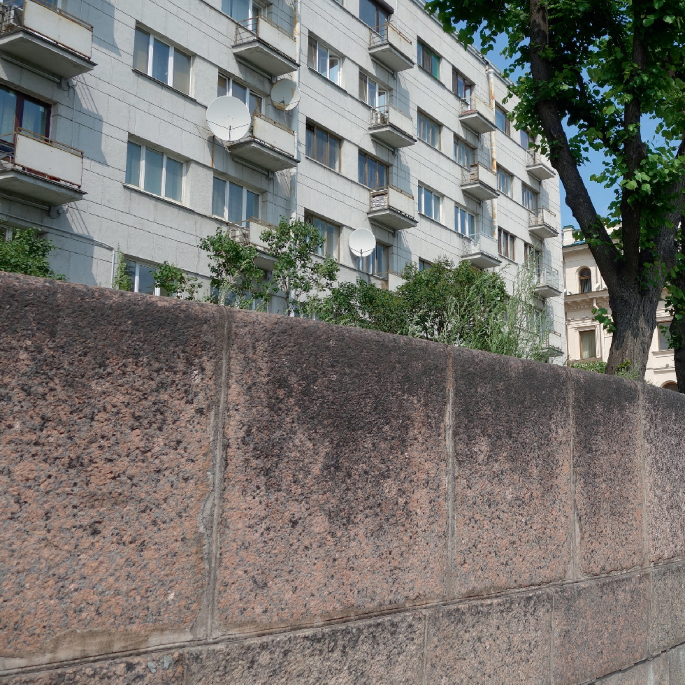This photo showcases a white or pale gray apartment complex with five visible stories. Each level features two windows per apartment, totaling in three windows each. Small balconies extend from each apartment, many equipped with satellite dishes. Just below the balconies, there is a dirty, old concrete wall composed of square stone blocks that are showing signs of age and discoloration, particularly towards the top. In the foreground, green trees stand in front of this wall, adding a touch of nature to the image. An additional building is partially visible on the right edge of the photograph. There are no people pictured in this scene, which emphasizes the architectural and natural elements.